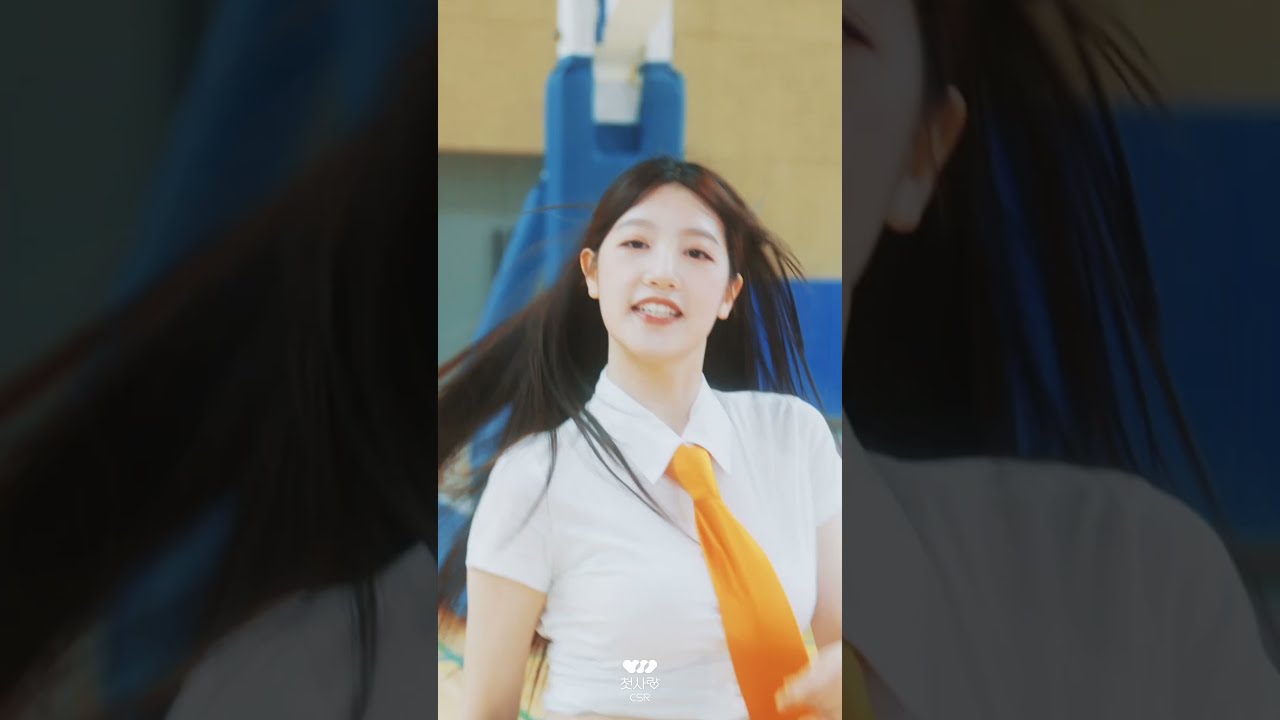The photograph captures a young Asian woman with long, straight black hair and dark eyes, wearing a white short-sleeved button-down collared shirt accompanied by an orange tie. She is smiling and appears to be looking directly at the camera, with her shoulders slightly turned as if responding to someone calling her name. She is also wearing earrings. The setting appears to be a gymnasium, indicated by the background elements which include a tan-orange wall, a large blue and white piece of sporting equipment that likely belongs to a basketball hoop, and a light blue door. The image, which seems to have been taken from a TikTok or Instagram Reel, is cropped in such a way that it magnifies her face and hair while fading out the sides, with only part of the right side of her face and left side of her hair visible.